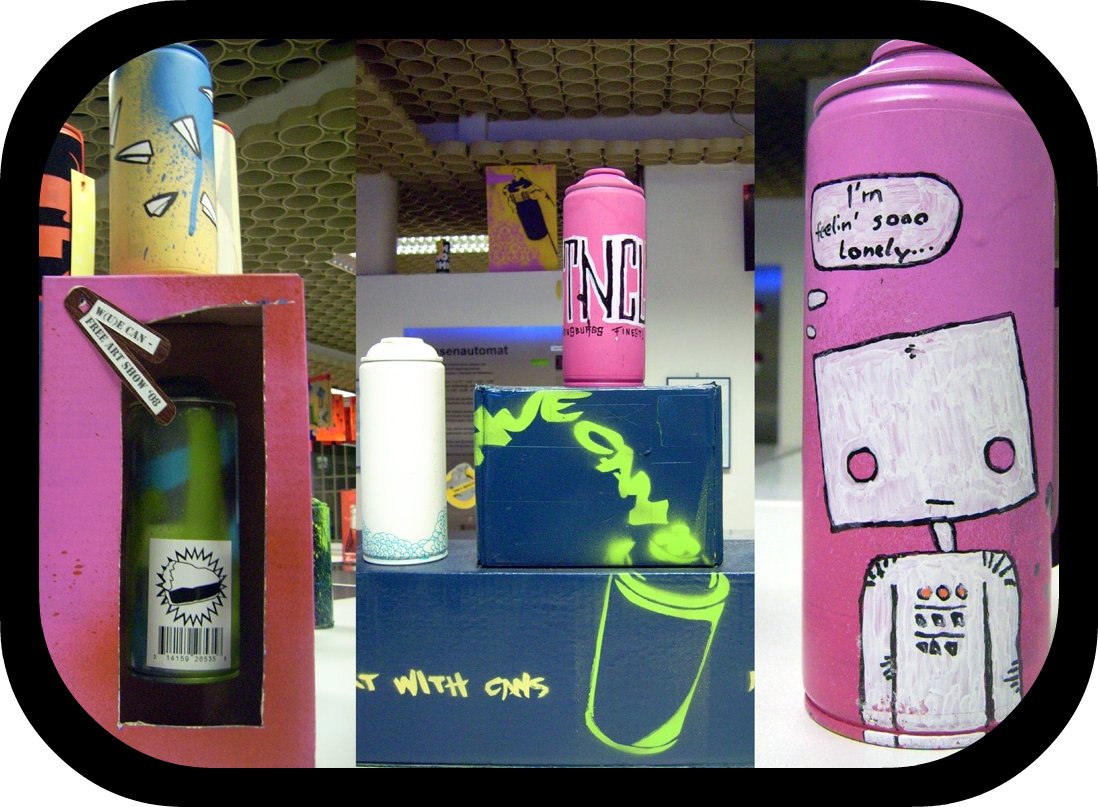This photograph showcases an art installation divided into three vertical segments, each within a rounded rectangle with a thick black border. Each segment provides a detailed glimpse into various components designed to mimic graffiti art.

In the left segment, a bright green spray can sits atop a tall pink box, which has a cutout revealing another can inside it. The inner can features green and blue lines with a spiky circle, and a barcode at the bottom. Two brown tags on this box read "white can" and "free art show 08."

The middle segment displays two stacked, blue-painted cardboard boxes: a wider one on the bottom and a smaller, more square one on top. A white spray can with blue bubbly patterns sits atop these boxes, and yellow text positioned on the boxes reads "with cans," though a preceding letter cut off with a T remains obscured.

In the right segment, we see a close-up of a pink spray can decorated with a sad robot design and thought bubble text stating, "I'm feeling so lonely..." Additionally, a yellow can at the bottom exhibits blue spray paint drips and doodles of paper airplanes.

The comprehensive view blends these eclectic elements into a cohesive and vibrant art piece, capturing an urban aesthetic with detailed layers of graffiti-inspired artwork.